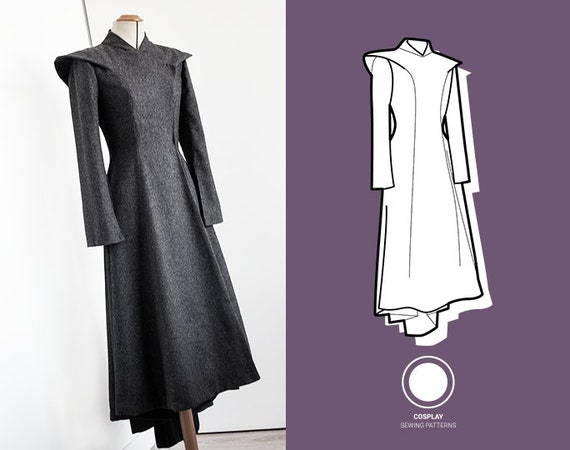The image showcases two visuals side-by-side: on the right, a graphic design of a black-and-white dress pattern set against a purple backdrop with a solid white circle at the bottom, labeled "Cosplay Sewing Patterns." On the left, a photograph depicts the actual dress, now realized as a mid-calf length, gray woolen one-piece with long sleeves and pronounced shoulder pads. The dress is displayed on a simple, headless mannequin with a stick-like support. This detailed comparison highlights the transition from the conceptual drawing to the tangible garment, demonstrating the pattern’s practical application.